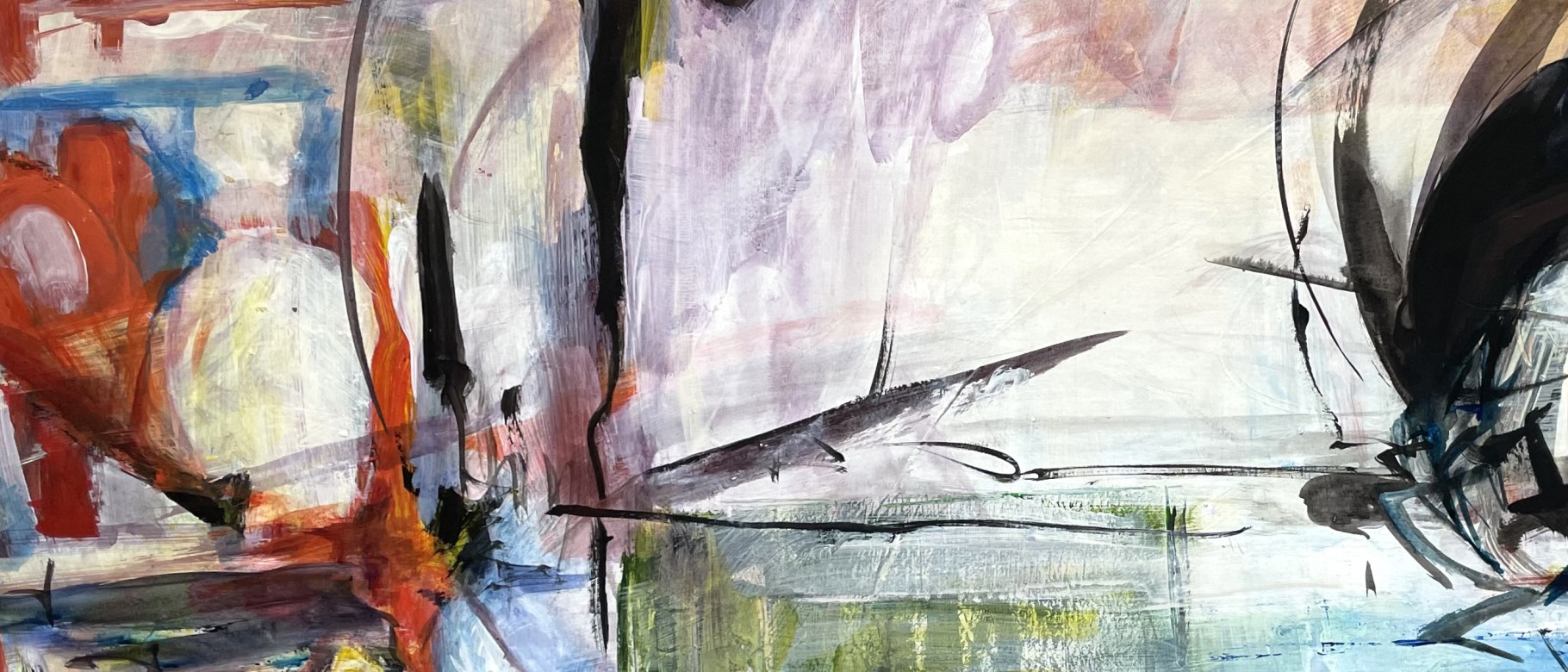The image is a photograph of a rectangular oil painting on canvas, characterized by its highly abstract nature. The top and bottom sides of the painting are significantly longer, almost two to three times the length of the left and right sides. The composition features a variety of colors and shapes distributed irregularly across the canvas.

On the right side, there's a distinct red oval shape with a smaller purple shape on top. Adjacent to these, a white circle shape is noticeable. Above these shapes, three blue lines form a structure reminiscent of a house. To the right of this, there's a sequence of colored lines: red, black, followed by a mix of white and purple, contributing to the overall abstract feel of the piece.

Prominent black lines feature in the painting, one being a large line intersecting with a thinner line at a right angle at the center of the canvas. Below this intersection, a green square emerges, partially obscured by various streaks of green and white paint.

The background reveals light blue and grayish hues, particularly on the bottom right, with swathes of white dominating the central area and blending into other shades. Some observers note that the shapes and colors suggest abstract forms like a smudge of black paint, possibly depicting a figure or driver in a car on the left side, dressed in white and topped with a hat. Despite these interpretations, the artwork's abstract smudges and smears of color remain open to varied interpretations.